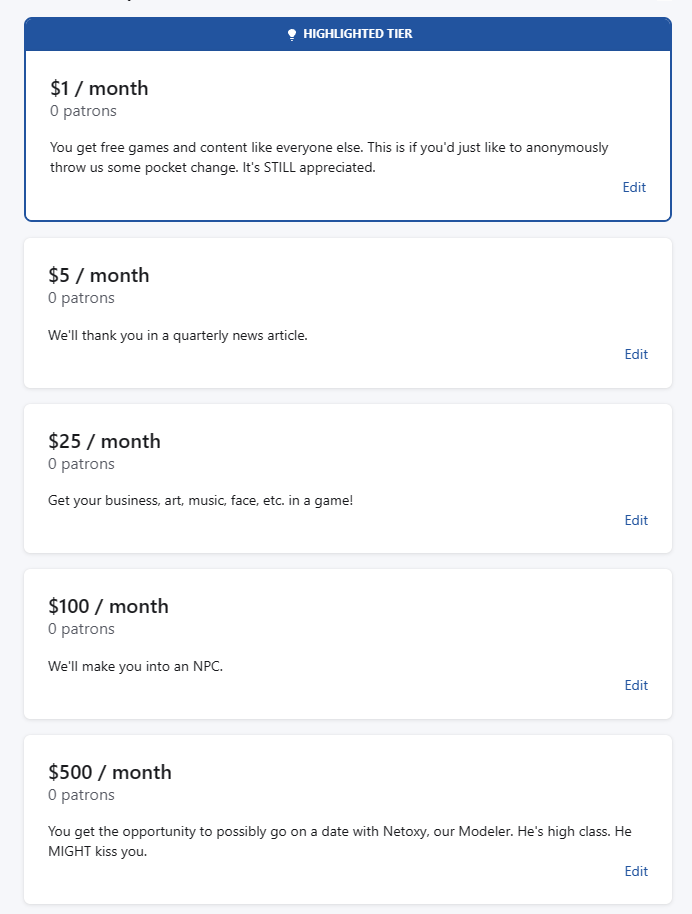The image depicts various tiers of a subscription model, each enclosed in a rectangular box with specific details:

1. **Highlighted Tier**: The box features a blue top border with the text "Highlighted Tier" in white. The rest of the rectangle is white and includes the text "$1/month, 0 patrons" followed by the description: "You get free games and content like everyone else. This is if you just like to anonymously throw in some pocket change. It's still appreciated." The word "still" is capitalized for emphasis. The bottom right corner has an "Edit" button in blue, bordered by a blue line.

2. **$5 Tier**: This white rectangle states "$5/month, 0 patrons" with the accompanying benefit: "We'll thank you in a quarterly news article." Similar to the previous tier, the bottom right corner has a blue-bordered "Edit" button.

3. **$25 Tier**: Another white rectangle indicating "$25/month, 0 patrons." The reward description reads: "Get your business, art, music, face, etc. in a game." An "Edit" button resides in the bottom right corner, bordered in blue.

4. **$100 Tier**: The white rectangle displays "$100/month, 0 patrons" with the description: "We'll make you into an NPC (Non-Playable Character)." The "Edit" button is again located in the bottom right corner with a blue outline.

5. **$500 Tier**: This last white rectangle outlines "$500/month, 0 patrons." The unique benefit for this tier is: "You get the opportunity to possibly go on a date with NETOXY or Modeler. He's high class. He might kiss you." The bottom right corner shows the "Edit" button, bordered in blue.

Each tier displays a consistent design, with the subscription price and the number of patrons prominently shown, followed by a detailed description of the corresponding benefit. All have an "Edit" button in the bottom right corner for customization.